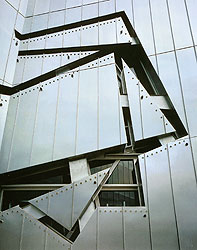The image is a vertical rectangular photograph of the side of a modern, multi-story building with a strikingly abstract and geometric design. The exterior features large, vertically arranged metal panels with intricate cutouts and jagged lines, giving the building a dynamic, almost fragmented appearance. The metal panels, predominantly gray, create triangular shapes bolted into the surface, enhancing the modern aesthetic. Set behind these panels are glass windows framed in lighter gray or silverish metal. One prominent window, positioned slightly above the bottom left corner, features a horizontal rectangular shape with a white plank running through its center. Above and around this window, additional cutouts in the wall form complex geometric patterns, including vertical and horizontal rectangles and thin triangles, further contributing to the building's unique architectural style. The overall color scheme comprises varying shades of gray, reinforcing the contemporary and minimalist vibe of the structure.